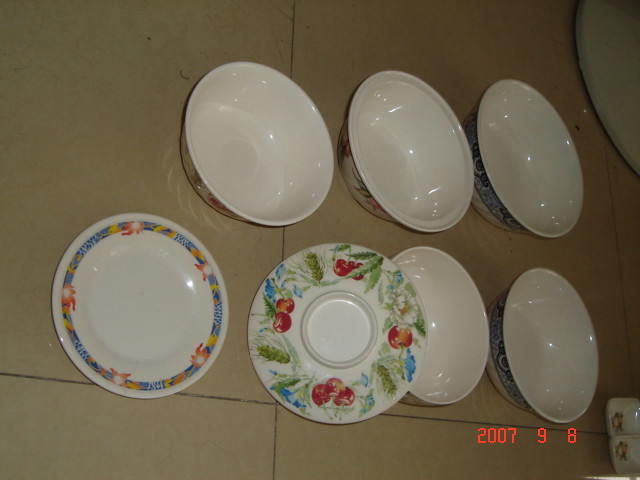The image shows an assortment of ceramic dishware arranged on what appears to be a beige tiled surface, likely a table. The composition consists of two rows: the top row features three bowls, while the bottom row displays two plates flanked by two additional bowls. The bowls, which have plain white interiors, exhibit various decorative patterns. Some bowls feature floral designs with pink and green hues, while others showcase an intricate blue and white pattern. The plates also boast distinct designs; one plate has a blue, pink, and yellow patterned rim, and the other displays a design of red cherries and blue flowers intermixed with green leaves, possibly a saucer given its central indentation. In the bottom right corner of the photograph, an orange timestamp reads "2007 9 8," marking the date.